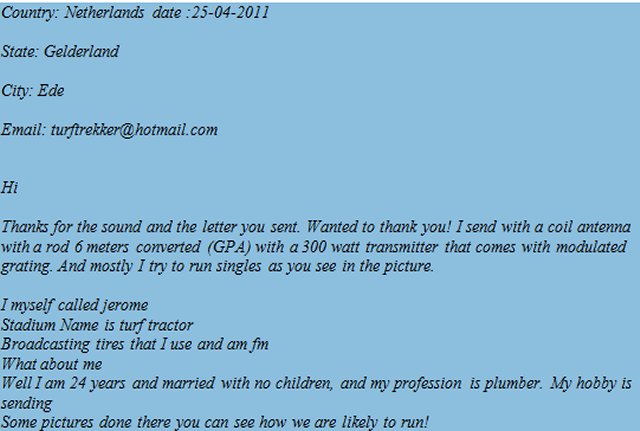The image is a landscape-oriented excerpt from an email, featuring a light periwinkle blue background with small italic black font. In the upper left-hand corner, it lists "Country: Netherlands" and the date "25-04-2011." Below this, it provides additional details: "State: Gelderland," "City: EDE," and "Email: turftrekker@hotmail.com."

The body of the message begins with a greeting: "Hi, thanks for the sound and the letter you sent. Wanted to thank you. I send with a coil antenna with a rod 6 meters converted with a 300-watt transmitter that comes with modulated grating. Mostly, I try to run singles, as you see in the picture. I myself am called Jerome. Stadium name is Turf Tractor. Broadcasting tires that I use are FM. What about me? Well, I am 24 years old, married with no children, and my profession is plumber. My hobby is sending pictures so you can see how we are likely to run."